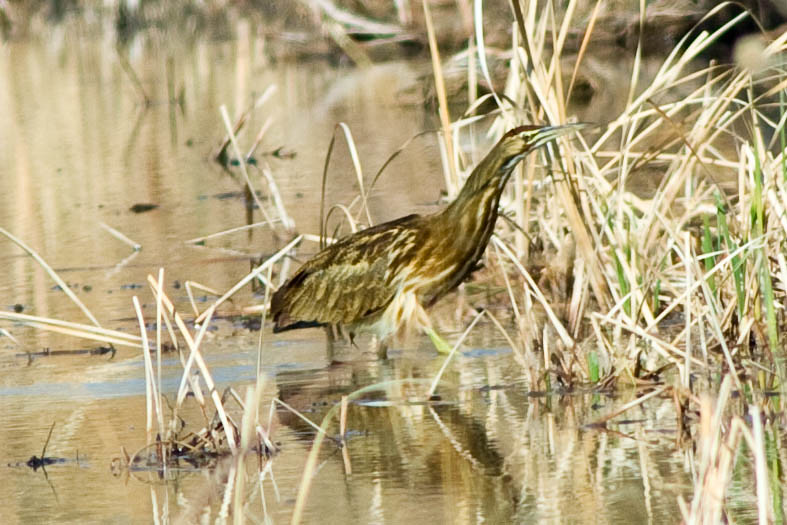This is a horizontal rectangular, full-color photograph taken outdoors during the daytime, capturing a swampy landscape dominated by rich brown hues. In the center of the image stands a sleek bird, cloaked in various shades of brown, blending seamlessly with its surroundings. The bird features a sharp, pointed beak and legs submerged in the water, which has a shiny surface interspersed with clusters of brown weeds. The bird appears to be gazing intently through the dense weeds, perhaps searching for prey. In the background, additional elements like rocks or logs are faintly visible along the distant shore, adding texture to the scene. Though predominantly brown, hints of blue in the water and a touch of green grass on the far right break up the monochrome palette, creating a captivating natural tableau.